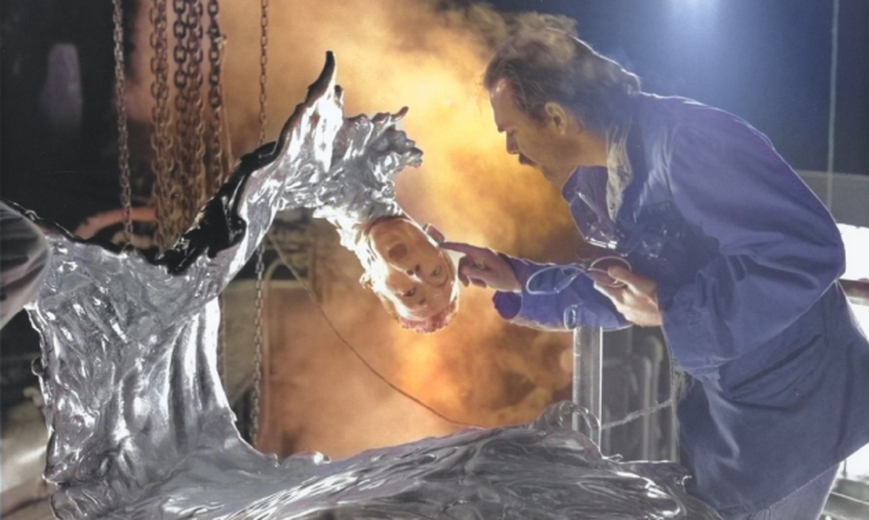This detailed photograph appears to be a behind-the-scenes still from a movie, possibly a scene in the foundry from "Terminator." On the right side, a man with a mustache, dressed in a blue jacket, and sporting slightly longer hair, is leaning over towards the centerpiece of the image. He holds a visor-like device in one hand while his other hand touches the ear of an intricate silver sculpture. The sculpture resembles a wave starting flat at the bottom, curving to the right, and turning into melted metal with a human head at the crest. The head, complete with open eyes, nose, and mouth, appears inverted and has light-colored hair, symbolizing a liquefied body. In the background, several chains hang from the ceiling amidst billowing, fiery orange-yellow smoke, adding to the dramatic and intense atmosphere of this cinematic moment.